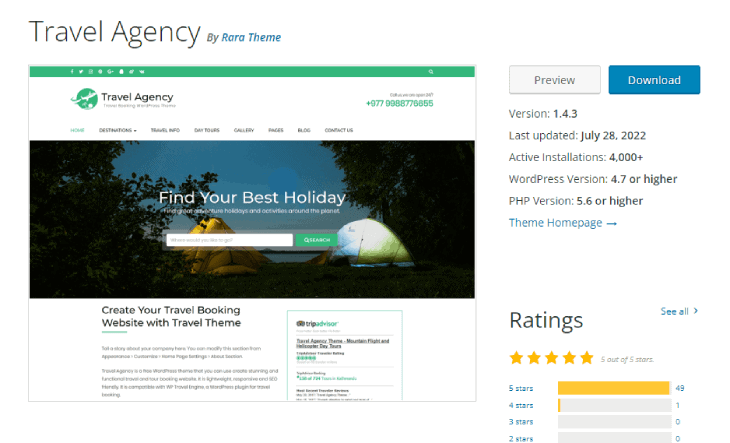In the upper left corner of the image, black text reads "Travel Agency by Rara Feen" ("Rara" spelled R-A-R-A). At the center, a green circle with an airplane icon holds the text "Travel Agency" and the phone number "977-9988-776-655." Below this, several subcategories are listed: Media, Notes, Pages, Blog, Contact Us, and Home, with "Home" highlighted in green text. 

The backdrop features a nighttime scene with a starry sky. In the foreground, there are two illuminated tents, surrounded by distant trees. The text "Find Your Best Holiday" overlays the scene, promoting the travel agency's message. 

Further text states "Create Your Travel Booking Website with Travel Theme," alongside a 5 out of 5 star rating from TripAdvisor. To the right, a detailed review section shows "49 5-star reviews" with the text "Version 1.4.3," indicating the product was last updated on July 28, 2022. It notes "Active Installations 4000+" and requires "WordPress version 4.7 or higher" and "PHP version 5.6 or higher."